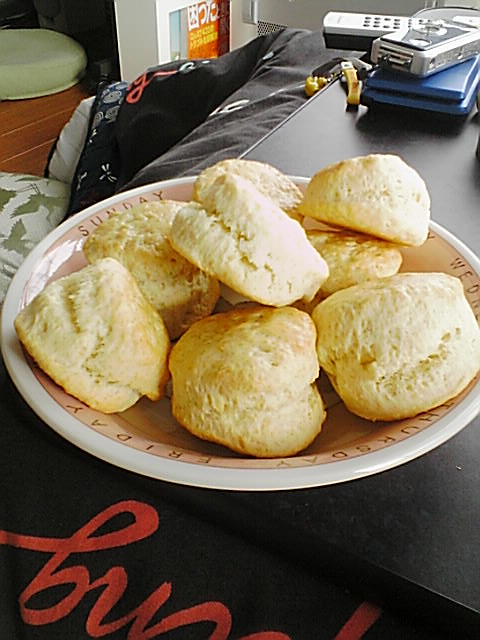This image depicts a plate of homemade biscuits, positioned on a wide white-rimmed bowl with a tan interior, which features the days of the week etched into it. The bowl, containing at least eight or nine lightly browned biscuits—with one prominently centered and stacked on the others—is placed on a black tray or table. A black pillow with red writing is partially visible beneath the bowl. Surrounding the setup, various items such as remote controls, possibly a wallet, a digital camera, and several cell phones are scattered around. The background reveals a cozy living area with a couch and a wooden floor, along with a white poster featuring red writing in an Asian language, which appears to be part of a book or divider.